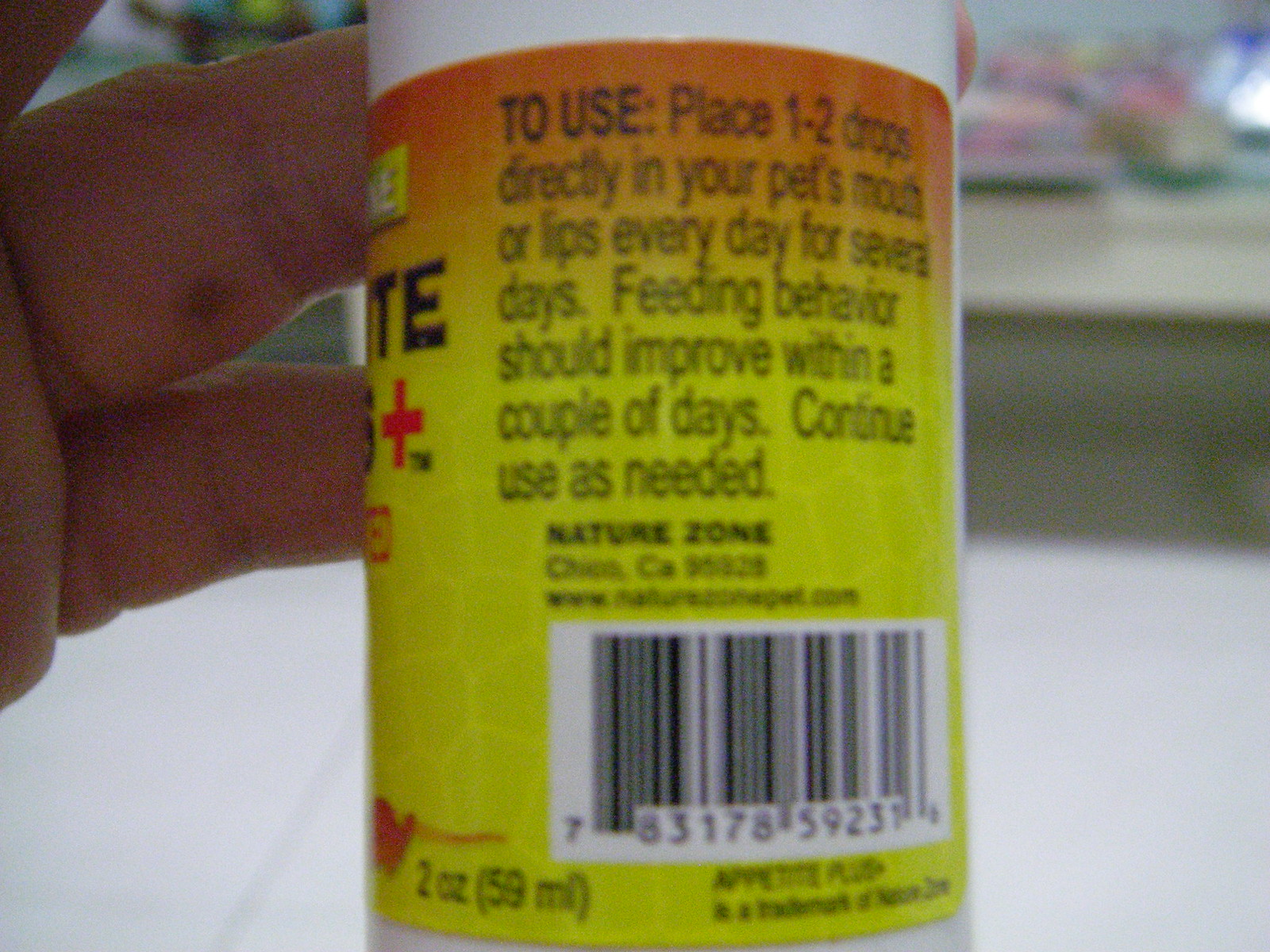In the image, a close-up shot captures a hand holding a small bottle of medicine. The bottle is predominantly yellow with a white lid and an orange ring around the cap. The clear text on the bottle's label provides specific usage instructions: "To use, place one to two drops directly into your pet's mouth or on their lips every day for several days. Feeding behavior should improve within a couple of days. Continue use as normal." Additionally, the label indicates the product is from Nature Zone, based in Chico, California. There is a black and white barcode, and although parts of the label, including the zip code and website (possibly naturezonepet.com), are too blurry to read, the overall appearance and information suggest it is a carefully designed medicine intended for pets.